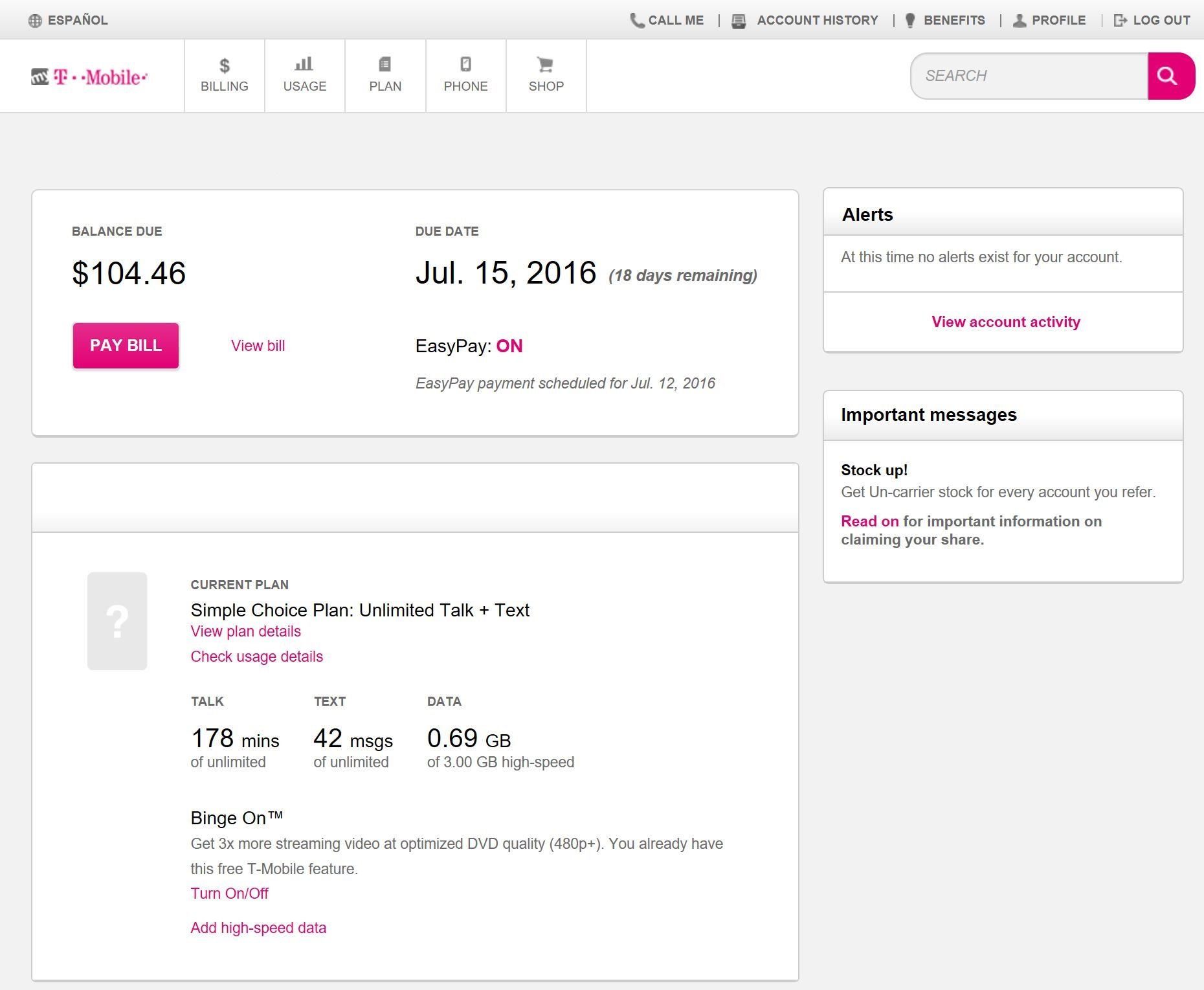**Detailed Caption:**

The image showcases the online account overview for a T-Mobile customer, displayed on a website with options in Spanish. At the top, the navigation menu includes links labeled "Call Me," "Accounting History," "Benefits," "People," and "Log Out." The T-Mobile logo is prominently displayed. Below the navigation menu, a horizontal white bar provides various options including "Billing," "Usage," "Plan," "Phone," and "Shop." A search bar is located on the right side for easy access.

The main section of the page prominently displays a billing summary within a rectangle. The current balance due is shown as $104.46, with a due date of July 15, 2016, and 18 days remaining to make the payment. A dark pink "Pay Bill" button is available for immediate payment, and there is also an option to "View Bill" in a similar color. To the right, it states that Easy Pay is enabled, with the next payment of $104.46 already scheduled for July 12, 2016.

There is an alerts section towards the middle, which currently shows no alerts, with a link to view account activities if desired. On the left side, details about the current plan are provided. The plan is named "Simple Choice Plan" and includes unlimited talk and text. There are clickable options to manage the plan, view plan details, and check the month's usage details, offering customers various ways to interact and manage their services with T-Mobile.